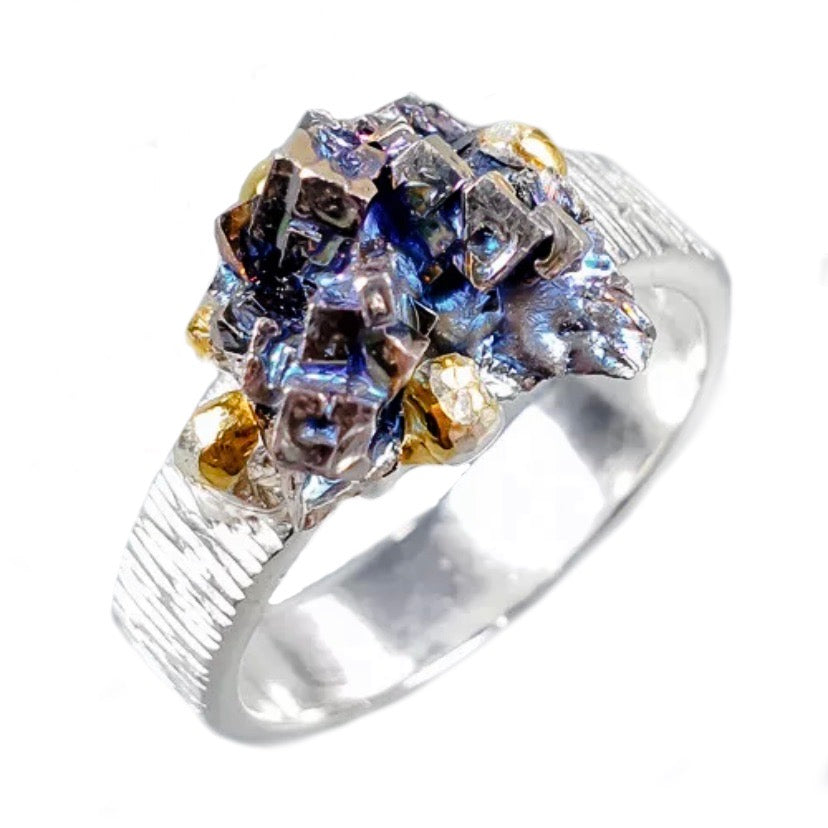This detailed close-up photograph of a ring showcases intricate craftsmanship and a unique design. The ring features a thick, silver band with a slightly bumpy texture, noticeable from the angle of the shot. The inside of the band is flat and shines with bright white spots due to the lighting. The focal point of the ring is an unusual stone formation on top, consisting of several smaller, cube-shaped stones fused together. These stones vary in color, displaying shades of yellow, gold, blue, purple, and metallic hues, creating a striking mosaic. The ring is set against a plain white background, highlighting its intricate details and vibrant colors. The image, taken at an approximate 45-degree angle, reveals both the top jewel portion and the inner band, providing a comprehensive view of this elaborate piece.